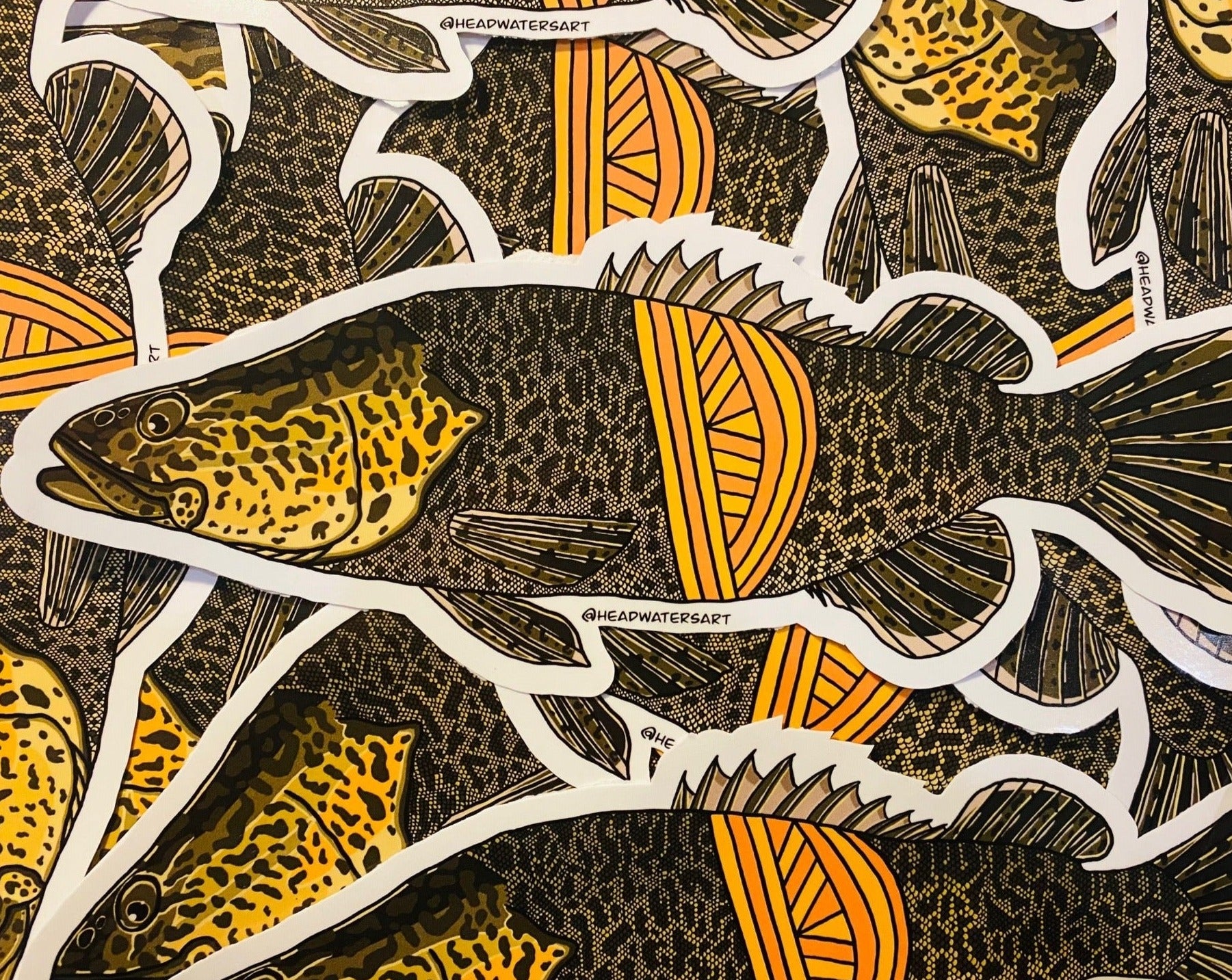The image showcases a hand-drawn, computer-generated fish, which appears to be part of a collection of overlapping stickers. The fish is primarily black and gray with intricate scales, accented by vibrant yellow and orange stripes along its midsection, giving it an apron-like appearance. Its head features a green face with a yellowish tint, and distinct eyes, with one visible brown eye containing a black pupil. The fish’s mouth is partially open. The fins, especially the back fins, are detailed and slightly green with a pointy appearance. Each sticker has a white cutout border and a copyright mark reading "Head Watersart." The stickers are layered haphazardly atop one another, suggesting a collage or a patterned assembly.